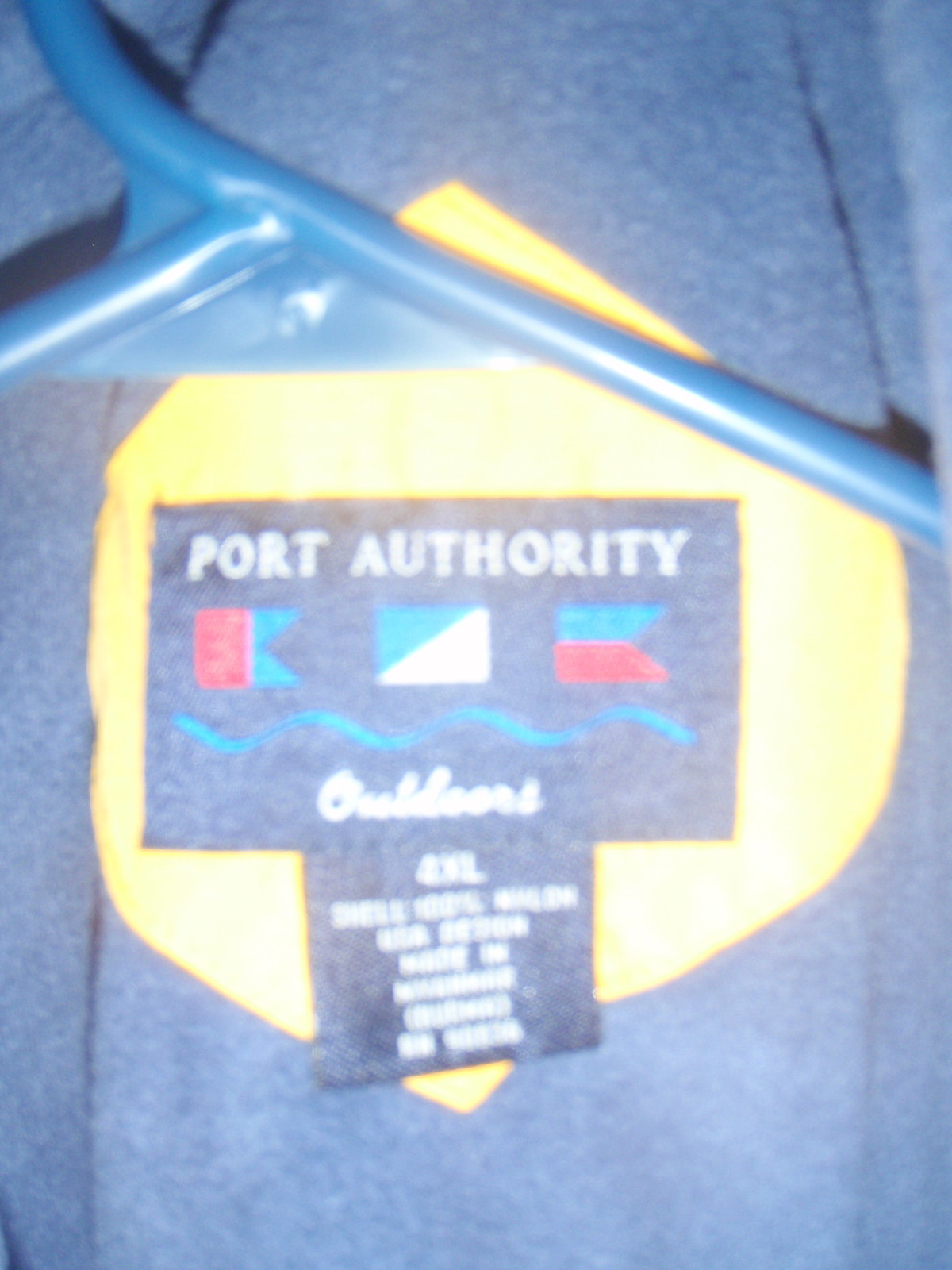This photograph captures a close-up view of a clothing label. The label is dark blue and rectangular, with "Port Authority" embroidered in white at the top. Beneath this text, there are several small flags; the central flag is turquoise and white, while the one on the right side is turquoise and red. A turquoise wavy line, resembling waves, appears below the flags. The text underneath this line is blurry, though it starts with an 'O' and may read "Outfitters" or "Outhouse." There is a smaller, square-shaped tag below, also dark blue with white writing, likely containing size and washing instructions, but it's difficult to decipher due to the blurriness. The fabric of the clothing item appears to be a medium blue fleece or fuzzy material and seems to be part of a shirt. An orange, almost yellow, circular shape is visible in the background. A blue plastic coat hanger is also partially visible at the top of the image.